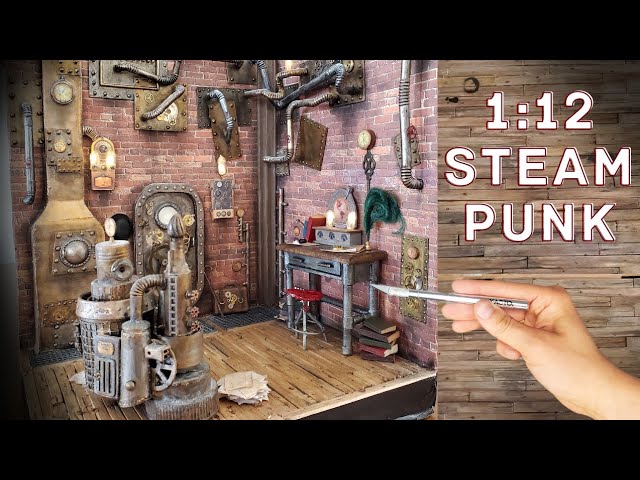The image showcases a detailed thumbnail or advertisement for a model building guide, specifically focusing on creating a 1:12 scale steampunk-themed room. On the right, white text with a red border reads "1 to 12 steampunk scale." The focal point is a hand holding a silver-handled X-Acto knife, poised in front of a small, meticulously crafted miniature wall designed with wooden planks. To the left, a richly detailed steampunk-themed scale model room features an intricate array of pipes and steam-powered machines adorning wooden floors and brick walls. A ship-like door enhances the theme, complemented by numerous devices, including clocks and unique apparatuses with pipes weaving in and out of the walls. Additional details include a table with a red stool, a stack of five miniature books, a box, and a scroll pen with a feather, hinting at a narrative depth and functionality within this captivating miniature world.